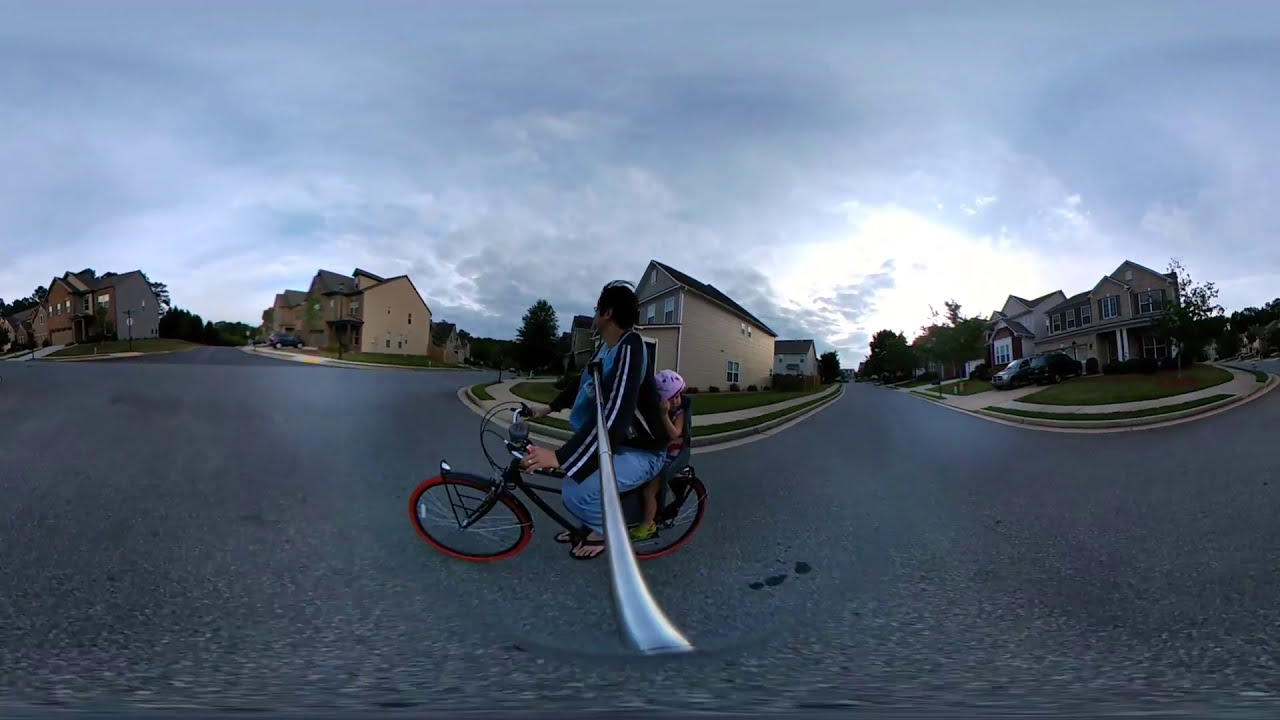The photograph depicts a horizontal, rectangular image of someone riding a bicycle on a dark gray paved road in a neighborhood with multi-storied tan houses that have triangle-shaped roofs. The rider, who has black hair and is possibly a woman, is dressed in jeans and a soft blue shirt beneath a black jacket with white stripes along the arms. The bike features dull red tires and appears to be black. Notably, there is a metallic selfie stick extending from the rider, seemingly attached to their chest, which also supports a long sword strapped across their back. Accompanying the rider is a child in a pink helmet seated behind them. The day is overcast with a mostly cloudy sky, casting a dark, illuminated ambiance over the scene as the houses dot the background with cars parked in some of their driveways.